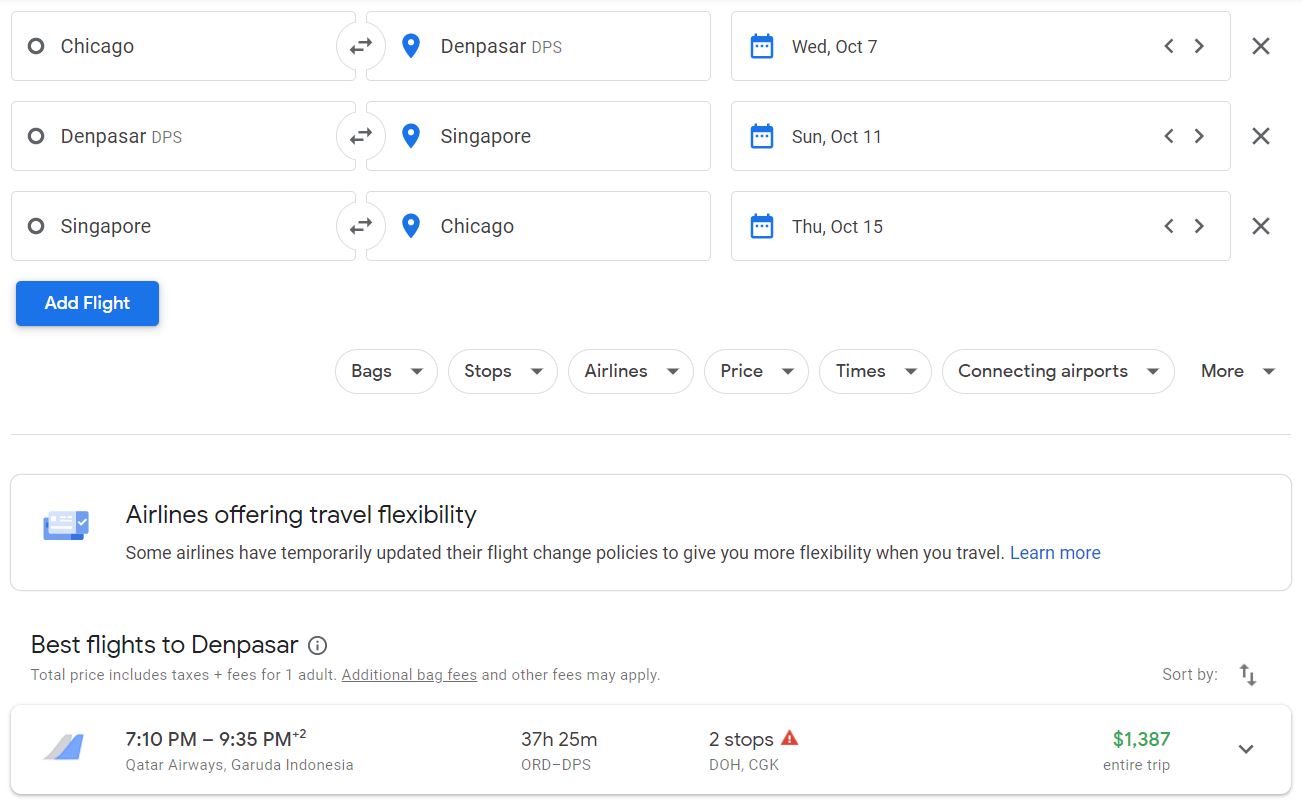This screenshot appears to be from a flight booking website, potentially for Qatar Airways. The top part of the screenshot is cut off, so the URL is not visible. The image displays a list of flights with the following details for each:

- **First Flight:** 
  - Route: Chicago (ORD) to Denpasar (DPS)
  - Date: Wednesday, October 7th

- **Second Flight:** 
  - Route: Denpasar (DPS) to Singapore (SIN)
  - Date: Sunday, October 11th

- **Third Flight:** 
  - Route: Singapore (SIN) to Chicago (ORD)
  - Date: Thursday, October 15th

Below these entries is a blue "Add Flight" button. Further down, there are filter dropdowns for refining the search results. These filters include:

- Bags
- Stops
- Airlines
- Price
- Times
- Connecting Airports
- More options

A gray line separates these filters from another section which has a gray rectangle box. This box contains information about airlines offering travel flexibility, mentioning that some airlines have temporarily updated their flight change policies to provide more flexibility. There is also a "Learn more" hyperlink in blue.

Beneath this information is a header titled "Best Flights to Denpasar," accompanied by an information icon. Below this header, small gray text states that the total price includes taxes and fees for one adult, mentioning that additional baggage fees and other charges may apply.

Lastly, there is another rectangle detailing a specific flight:
- Time: 7:10 PM to 9:35 PM (indicating a duration of 37 hours and 25 minutes, including two stops)
  - Airlines: Qatar Airways, Garuda Indonesia
  - Route: ORD to DPS
  - Stops: DOH (Doha), CGK (Jakarta)
  - Price: $1,387